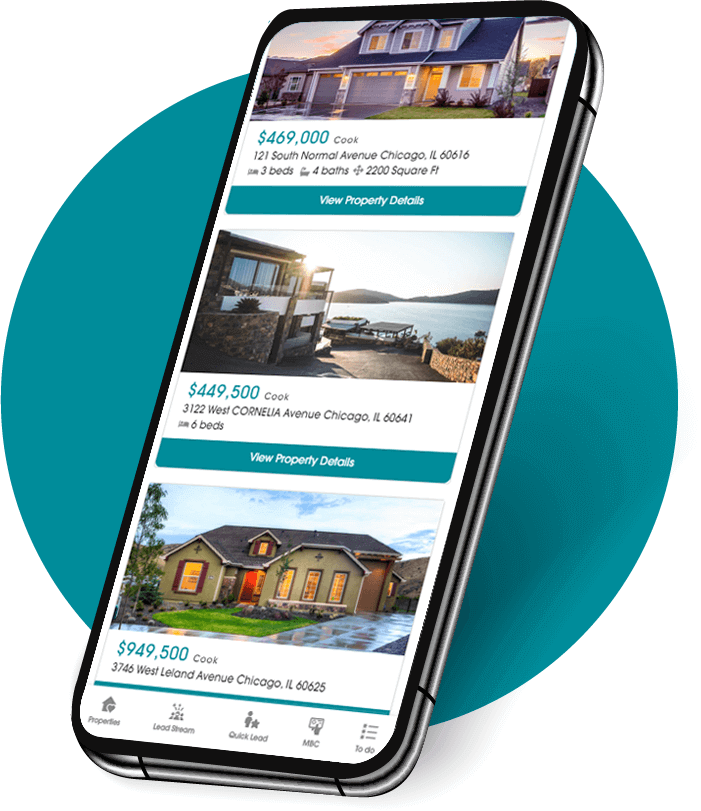This image appears to be an advertisement for a real estate app. The background features a vibrant turquoise blue circle. Dominating the foreground, a sleek black or silver smartphone is positioned diagonally from the bottom left to the top right, displaying what seems to be a house-buying app.

On the screen, several property listings are showcased:
1. The first listing features a charming, greyish double-story house with a sharply angled roof and three small windows at the top. This property, illuminated with lights from within, includes two garage doors and is listed at $469,000. Located at 121 South Normal Avenue, Chicago, it offers three bedrooms, four bathrooms, and spans 2200 square feet. The abbreviation "Cook" likely refers to its county. A blue tab on the screen invites viewers to "View Property Details."

2. The second listing presents a picturesque face brick house adjacent to a serene lake. Priced at $449,500, this property is situated at 3122 West Cornelia Avenue, Chicago, and boasts six bedrooms. A similar blue tab encourages viewers to view additional property details.

3. The final listing in the app highlights a lovely, avocado green-colored house within a neighborhood. While it appears to be a single-story home, there is a tiny room within the roof. The interior lights warmly illuminate this property, which is valued at $949,500 and located at 3746 West Leland Avenue, Chicago. This house also features a blue tab for viewing further property details.

Each listing provides vital information about the properties, catering to potential buyers seeking their dream homes in Chicago.